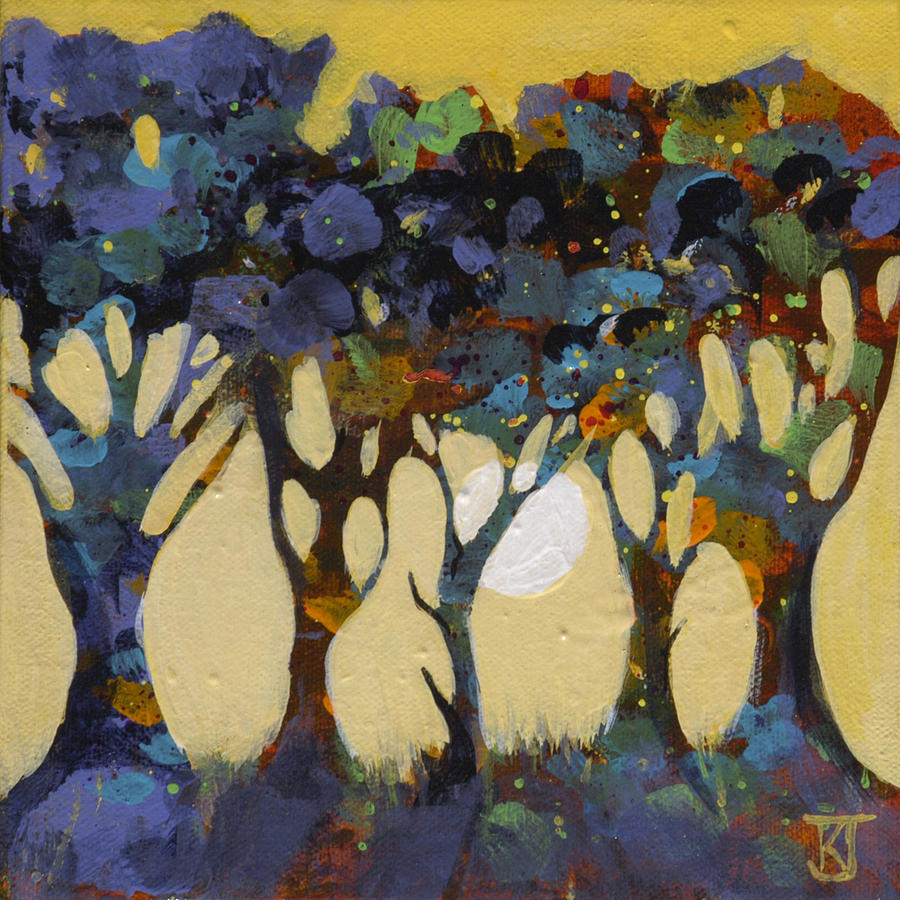This vivid oil painting features an intriguing array of colors and depicts an orchard-like scene with five evenly spaced trees against a contrasting and dynamic background. The top portion of the painting is dominated by dark and light shades of yellow, with a white circle centrally positioned, suggestive of the Sun. The middle section integrates a variety of colors, including green, purple, and darker hues like black, adding depth to the scenery. The ground is a vibrant mosaic of purple, brown, green, red, yellow, and orange spots. Each tree has distinctly colored trunks and leaves, showcasing mixtures of purple, teal, blue, brownish-red, green, yellow, and orange. The painting is signed with the initials 'KJ' in the bottom right corner. The colorful branches and leaves scattered across the canvas create a noticeable contrast, enhancing the overall vividness and beauty of the image.